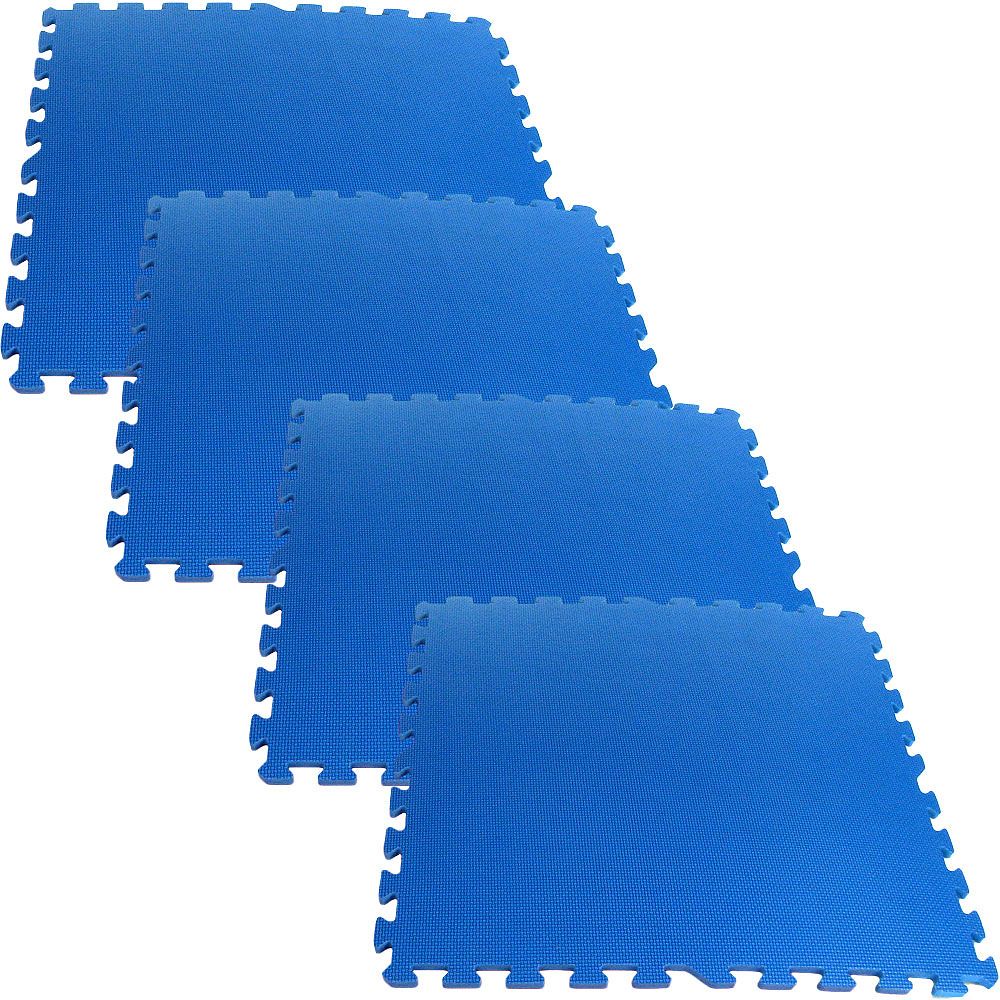This photograph showcases four medium blue, foam interlocking tiles arranged against a white background. These tiles resemble puzzle pieces with uniquely designed edges that include diagonals, allowing them to seamlessly connect. Each tile features a slightly textured surface, providing both visual interest and added grip. Despite appearing to vary in size due to their staggered and diagonal placement, these rectangular tiles are all uniformly sized, a visual trick that creates a 3D illusion. Ideally used for flooring, their soft foam composition ensures a cushioned surface, suitable for a variety of environments.